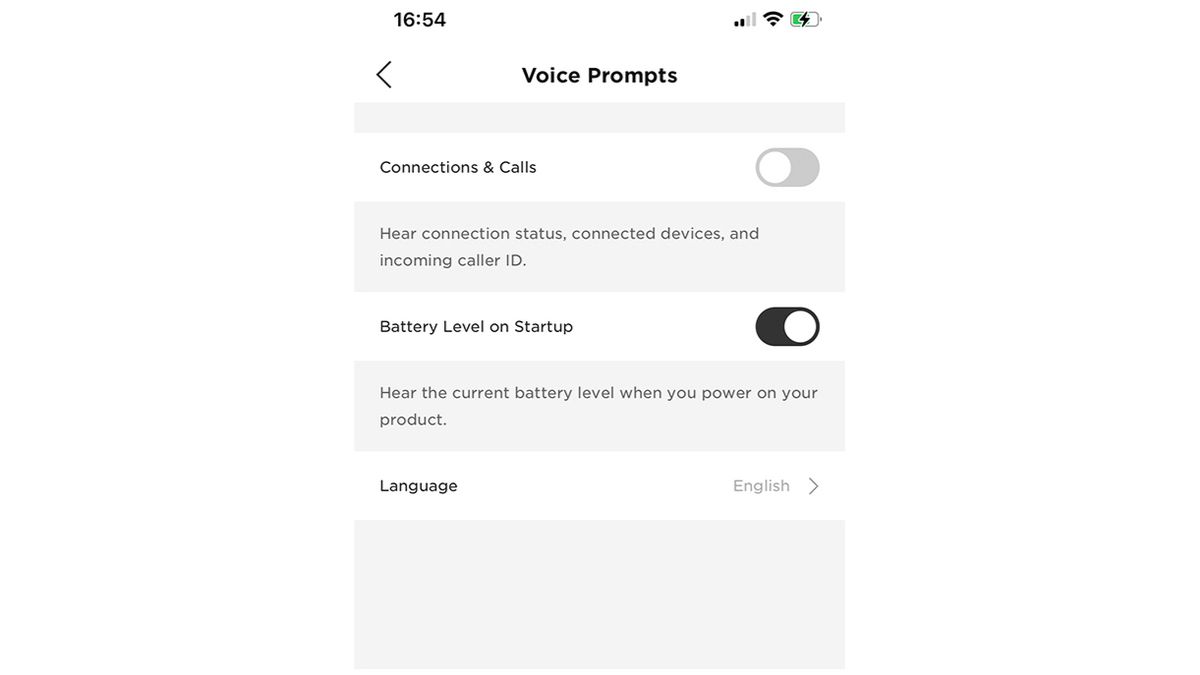The image is a tall, narrow screenshot from a cell phone displaying a settings menu. At the very top, the time reads 16:54 on the upper left, while the upper right shows both signal strengths and a battery at approximately 50%. Below, a navigation bar features a left back arrow; to its right, centered text in black states "Voice Prompts." A gray bar separates this from the next section.

Continuing down, the next area features left-aligned text "Connections and Calls" in smaller font. This option appears to be turned off, as indicated by a toggle on the right. The background here is a gray area containing a banner that reads "Connection Status," "Connected Devices," and "Incoming Caller ID." 

About 40% down, a white background section appears with left-aligned text "Battery Level on Startup," which is toggled on at the right. Further down, another gray background section explains, "The current battery level when you power on your product."

The following section has a white background with left-aligned text "Language." This text is bold, and on the right, dimmed in light gray, it reads "English" with a right-facing arrow. The bottom of the screenshot is capped by another gray bar.